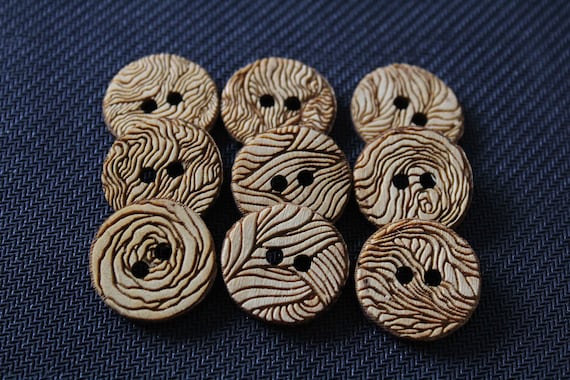The photograph depicts nine intricately designed wooden buttons arranged in a grid formation on a dark blue, diagonally-patterned fabric background. Each button, crafted from light beige wood with darker brown etchings, features a unique pattern resembling either small portions of fingerprints, tree bark, or floral designs viewed from above. The buttons each have two central holes and their distinct designs are captured in rich detail with none appearing identical. The buttons are slightly overlaid in such a way that they create a subtle angle, except for the back row, which is laid flat against the textured blue surface, enhancing the visual depth of the arrangement.